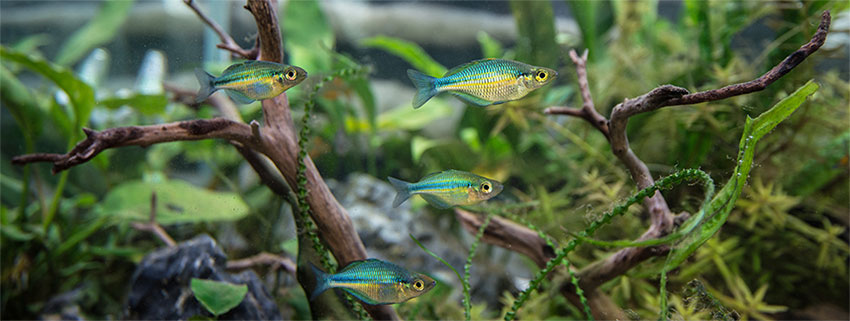This image appears to be the interior of a fish tank, although its edges are not visible, making it uncertain if it might actually be underwater somewhere. However, the remarkable clarity of the water suggests it is indeed a fish tank. At the center of the photo are four small, colorful fish. Three of these fish are staggered vertically, while the fourth swims to the left of the topmost fish. Each fish has a distinctive shiny coloration, with blue stripes on the top of their bodies and yellow underneath. Their eyes are detailed with a black pupil surrounded by a yellow ring.

Around the fish, the environment is richly detailed with aquatic vegetation, including seaweed and varieties of water plants. There are also elements of deadwood, with one stick prominently rising from the bottom right towards the top right and another stretching its branches towards the left. Scattered among these are rocks and some leaf matter, contributing to the naturalistic setting. Despite the absence of visible tank edges, the assortment of twigs, algae, and other underwater flora and fauna suggests a well-maintained, possibly sizable, aquarium habitat.